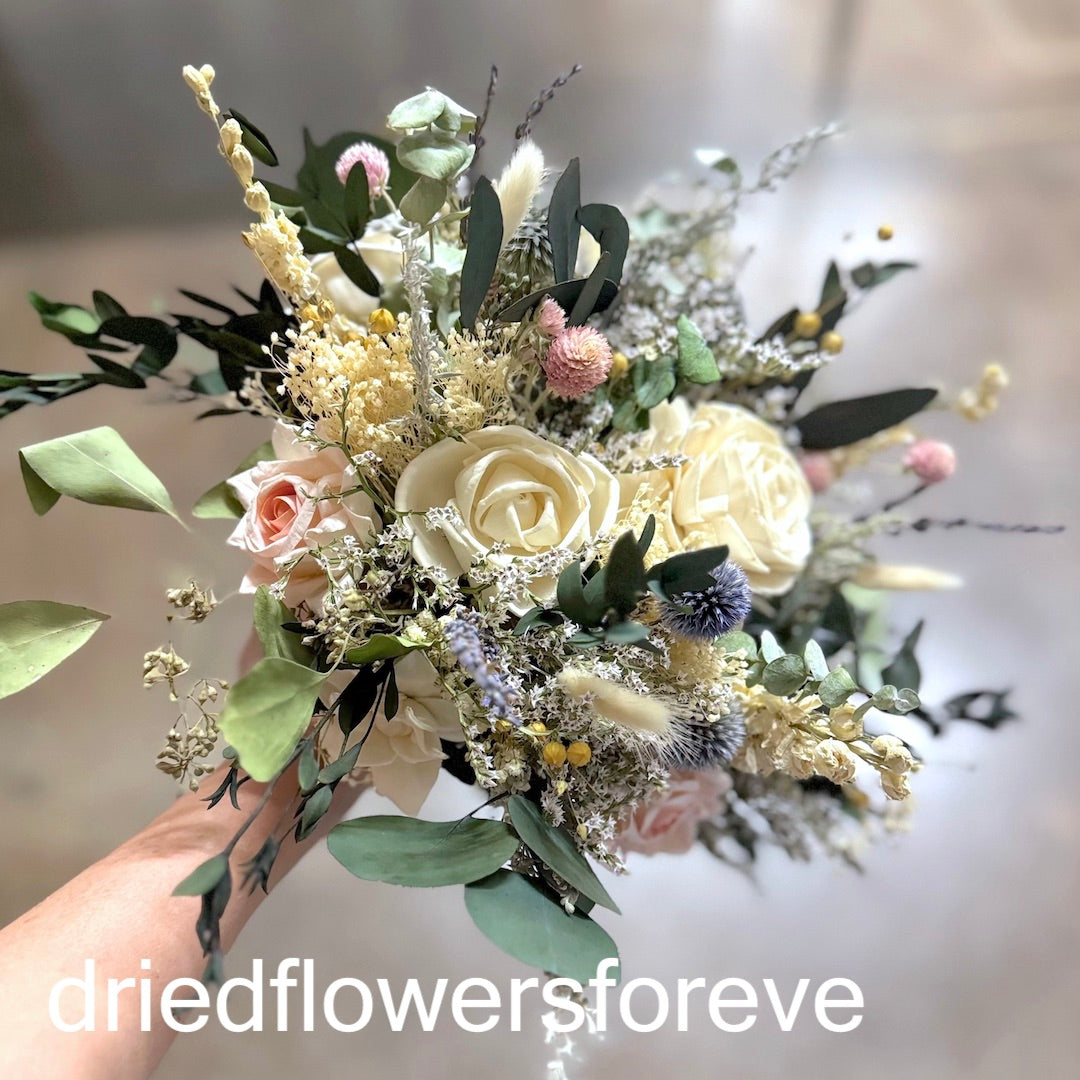In the image, an arm extends from the bottom left corner, holding a vibrant bouquet of dried flowers. The bouquet occupies most of the frame, showcasing a rich variety of colors and textures: pink and yellow roses, small white flowers, and green eucalyptus leaves. Additionally, there are blue spiky flowers, round yellow seed-like balls, baby's breath, and fuzzy elements interspersed among the blooms. The background is a hazy blend of light tan and gray, lending a soft, out-of-focus effect that highlights the bouquet. At the bottom of the image, white print reads "dried flowers for Eve."